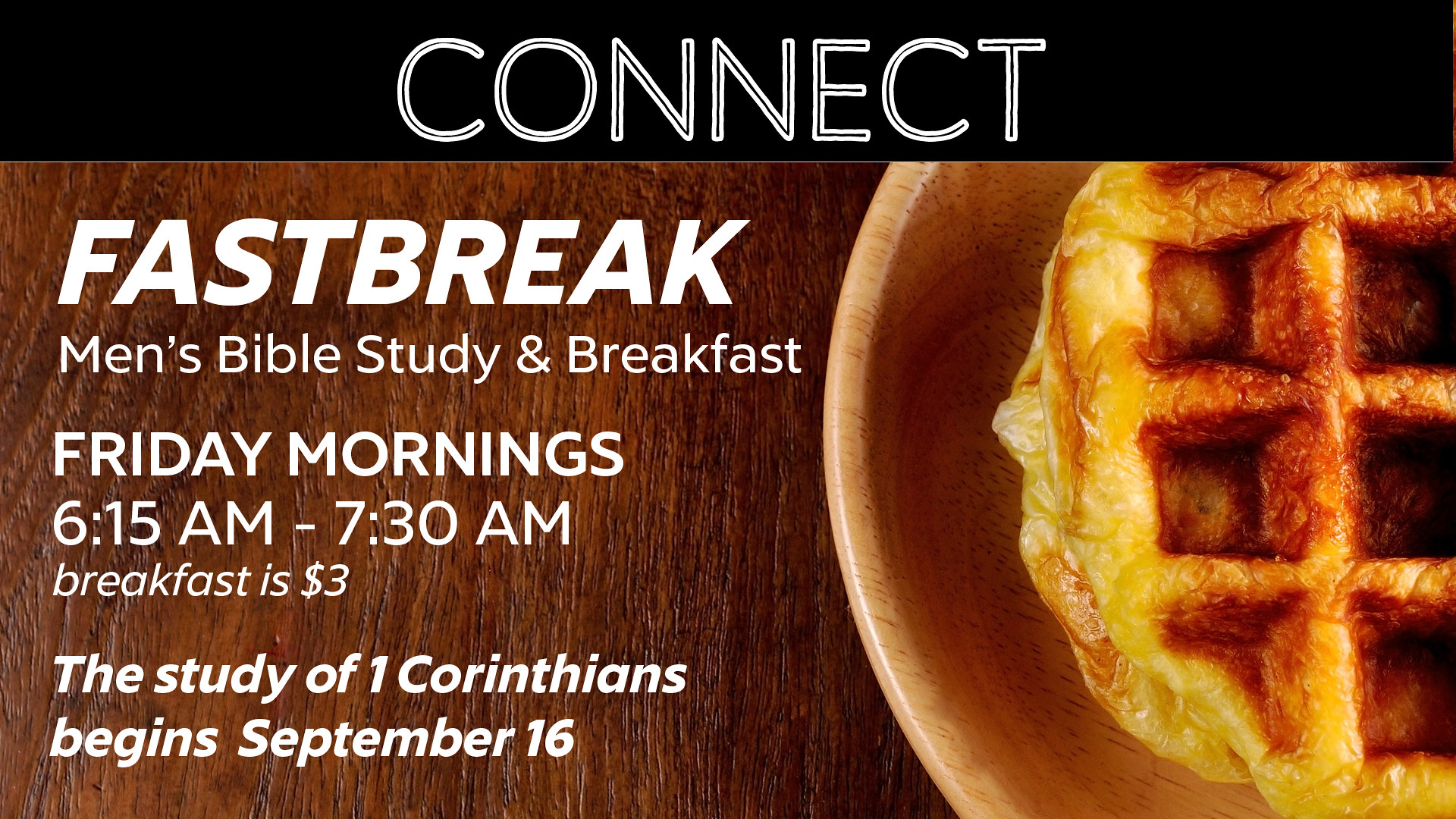The image is a scan or screenshot of an advertisement likely seen on social media, perhaps shared on a restaurant's Facebook page. The advertisement is divided into two sections. The top section features a thin black bar stretching horizontally across the image, with white text in all capital letters reading "CONNECT" at the center. Below that section, the bottom part of the image showcases a close-up picture of a wooden plate holding a waffle, set on a wooden table, creating a warm, earthy aesthetic with various hues of brown.

To the left of the waffle, which extends out from the right edge of the image, there is white text divided into several lines. At the top, it reads "FAST BREAK" followed by "MEN'S BIBLE STUDY AND BREAKFAST." Below that, it provides the details, "FRIDAY MORNING 6:15AM TO 7:30AM, BREAKFAST IS $3." The bottom two lines announce, "THE STUDY OF ONE CORINTHIANS BEGINS SEPTEMBER 16."